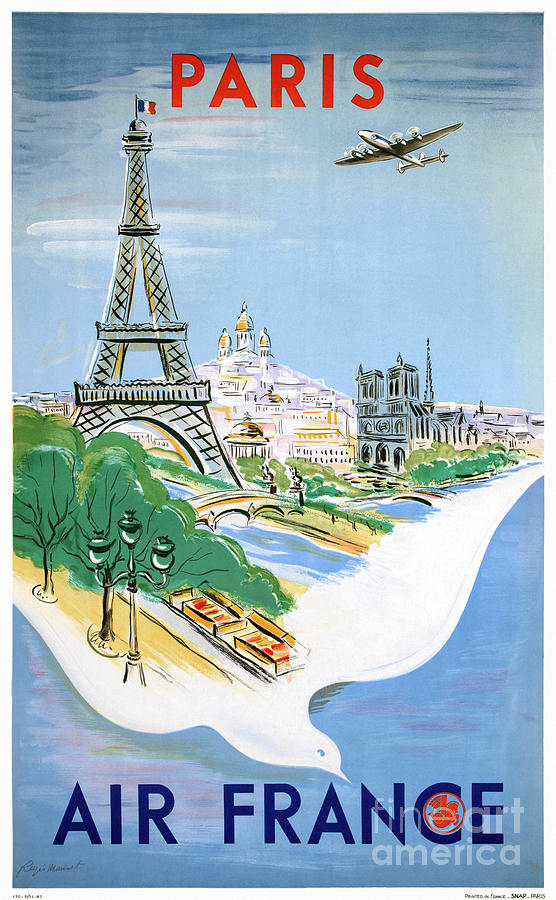This advertisement for Air France, seemingly the front of a pamphlet, features a vibrant, cartoon-style illustration of Paris. At the top, the word "PARIS" stands out in bold red capital letters, just above an old four-propeller airplane flying beneath the text. A picturesque and artistic depiction of Parisian landmarks dominates the center, with the Eiffel Tower and Notre Dame drawing immediate attention, supplemented by additional landmarks like gazebos and cityscapes in the background. The entire scene resembles a stylized map, accentuated by shapes and vivid colors. The map includes a flowing river, foliage, gray and white buildings, a bridge, and a park. A notable and imaginative detail includes a white bird or dove shape above the "Air France" text at the bottom, symbolizing elegance and freedom. The bottom of the image features the words "AIR FRANCE" in bold blue capital letters, with a blue ocean-like background transitioning upwards into a darker blue sky embellished with soft clouds. There is a watermark reading "Fine Art America" in the bottom right and an artist's signature in the bottom left, adding an artistic credential to this visually immersive and engaging advertisement.